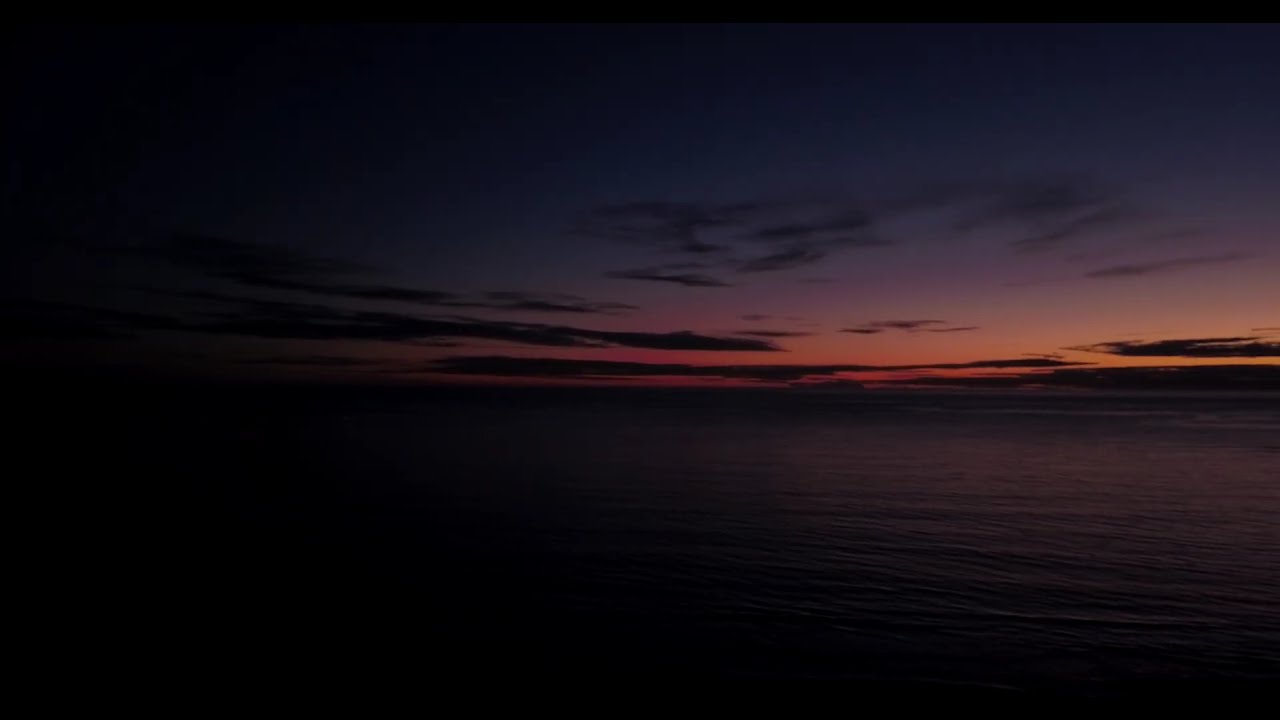The image depicts a tranquil seascape at dusk, captured just after the sun has set. The horizon line lies centrally, dividing the scene into a dark, calm expanse of water below and a richly colored sky above. The sky near the horizon glows with a vibrant blend of orangish-yellow, transitioning into pink, then to shades of purple, and finally to a deep blue higher up. Wispy stratus clouds appear scattered throughout the sky, silhouetted in black against the diminishing light. Towards the left, the scene fades into deeper darkness, obscuring details. The overall ambiance conveys a peaceful yet dramatic transition from day to night.